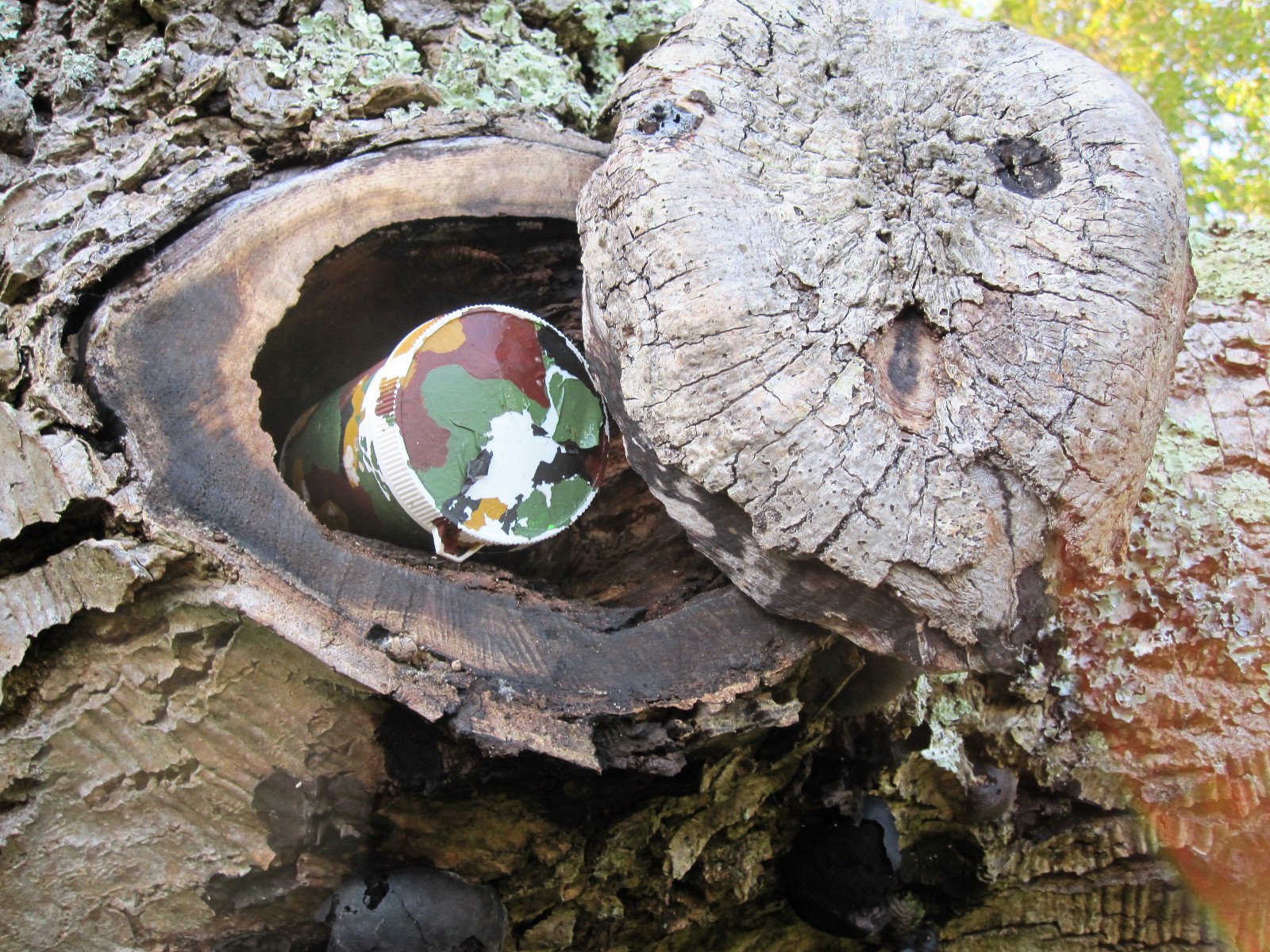The image depicts an outdoor scene in the woods featuring an old, rotted tree stump that has been cut and hollowed out, creating a hidden compartment. The top of the stump, which appears to be sawed off, has been shifted to the side to reveal the hollow interior. Inside this hollow space, there is a cylindrical, beat-up green camouflage canteen, resembling an old thermos or a tube for storing posters or blueprints. Surrounding the stump, there are hints of greenery, including some green, yellow, and white patches that suggest the presence of flowers or lawn grass, indicating it is daylight. The close-up view of the stump highlights the intricate details of this cleverly concealed hiding spot.